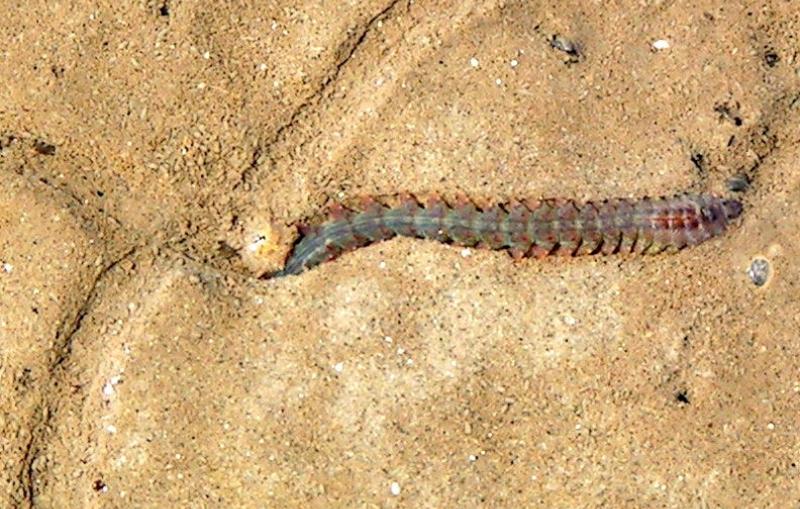In this detailed photograph, we see a centipede navigating a sandy terrain. The sandy ground, resembling a beach or dirt area, has a light tan to dark brown hue—indicative of moisture and possibly recent rainfall or proximity to a body of water. Small pebbles and grains of sand add to the texture of the scene. The centipede, partially submerged, displays a greenish body with a thicker, purplish-gray head adorned with brown flecks and reddish rings near the front. Sunlight shines down, highlighting the sandy texture and the centipede's segmented anatomy, which appears to be stationary, making it look almost like a part of the natural rocky formation surrounding it.